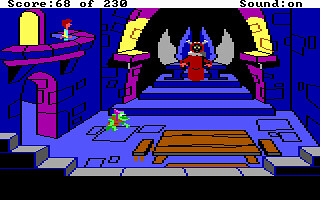This screenshot captures a pixelated, old-school video game scene set inside a dungeon-like castle with a blue-hued stone interior. The score displayed at the top reads 68 out of 230, with a "sound on" indicator also visible. Dominating the center of the image is a raised dais with three steps, upon which sits a throne backed by wings. Occupying the throne is a figure dressed in a red robe, featuring a black face with white eyes and possibly horns, suggesting a demonic or royal character. In the foreground, there's a wooden table and a gray brick wall that gives the sense of looking into the room.

A goblin-like creature, possibly a gremlin or a large frog, occupies the floor space near the throne, donned in an orange garment and pink hat, adding a whimsical touch. Additional details include a balcony area at the top left, where a person wearing a blue shirt and brown hair observes the scene. Light sources enhance the atmosphere: a purple light illuminates the left side of the balcony, casting a violet hue on the stone, while a yellow light also contributes to the color scheme, which prominently features shades of blue, purple, and yellow.